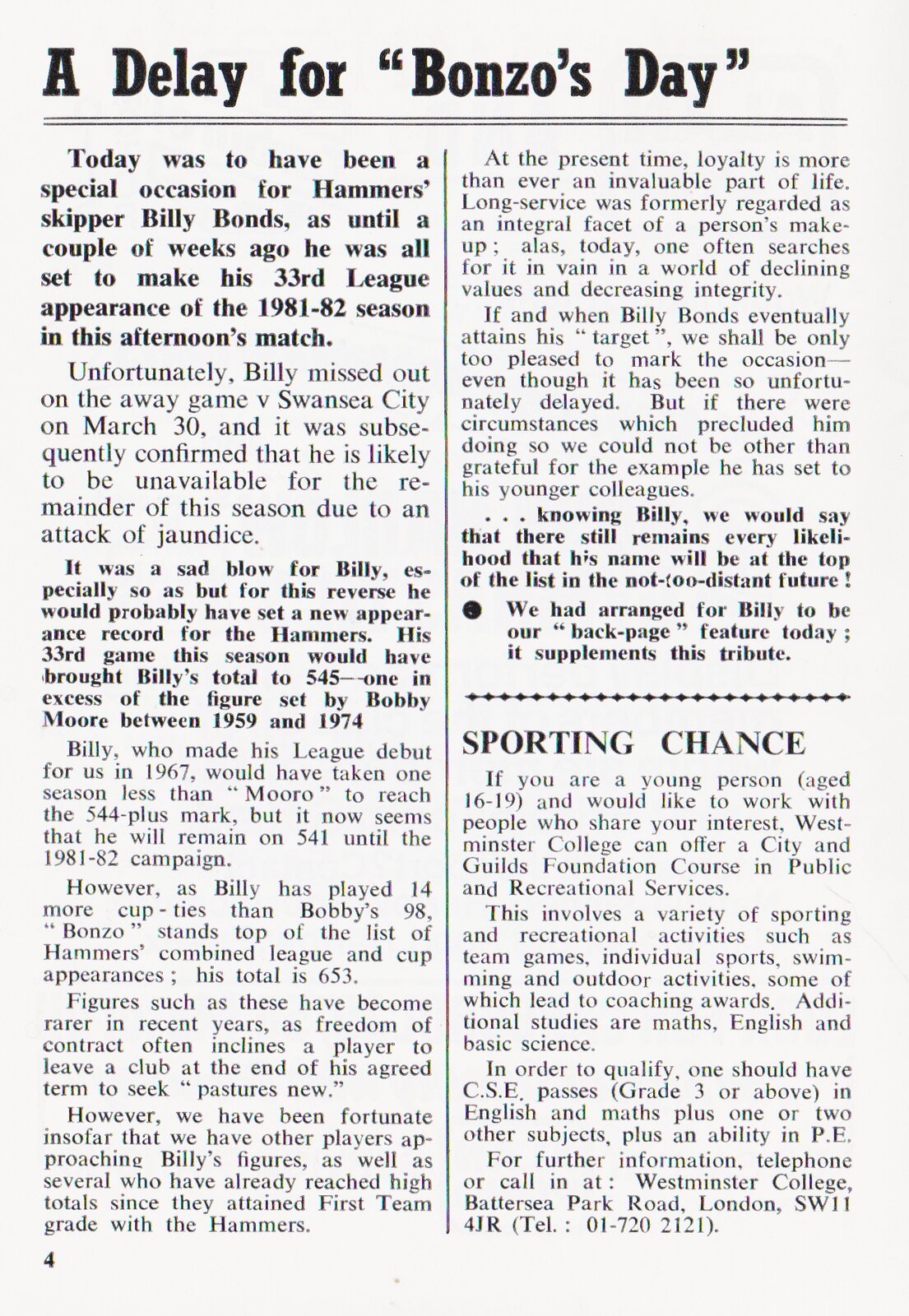The image is a detailed publication with a light grey background and black text, featuring an article titled "A DELAY FOR BONZO'S DAY" in bold dark black font at the top. Below the title, there are two parallel horizontal lines, and a vertical line divides the text into two columns. The left column consists of seven paragraphs, discussing the unfortunate circumstances surrounding Hammer Skipper Billy Bonds, also referred to as "Billy Bonzo," who, until recently, was set to make his 33rd league appearance of the 1981-82 season. The text elaborates on Billy's missed opportunity to play in the away game against Swansea City on March 30 due to jaundice, which likely rules him out for the rest of the season. This was a significant setback for Billy, as it hindered him from surpassing Bobby Moore's record of 544 league appearances, a record he was poised to break. The right column also contains seven to eight paragraphs, with sections in light and bolded font, including a smaller bolded paragraph highlighting the disappointment of Billy missing out on setting a new record, and emphasizing his outstanding contributions to the team. Additionally, there's a segment promoting a "Sporting Champs" course at Westminster College for young individuals aged 16 to 19, offering training in various sports and activities, which includes contact details for further information.